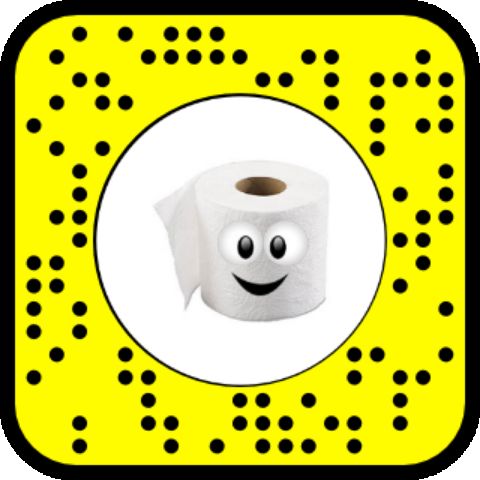The image appears to be a Snapchat icon featuring a yellow square with rounded corners, outlined by a black border and decorated with black polka dots around its perimeter. Inside this yellow square, there's a central white circle with a black border. Positioned within this white circle is a roll of toilet paper standing upright, with the brown cardboard tube visible at the top. The toilet paper roll is animated with a friendly face, characterized by two crossed eyes and a slightly open, smiling black mouth. This cheerful illustration and the icon's design hint at its association with an app or digital platform.